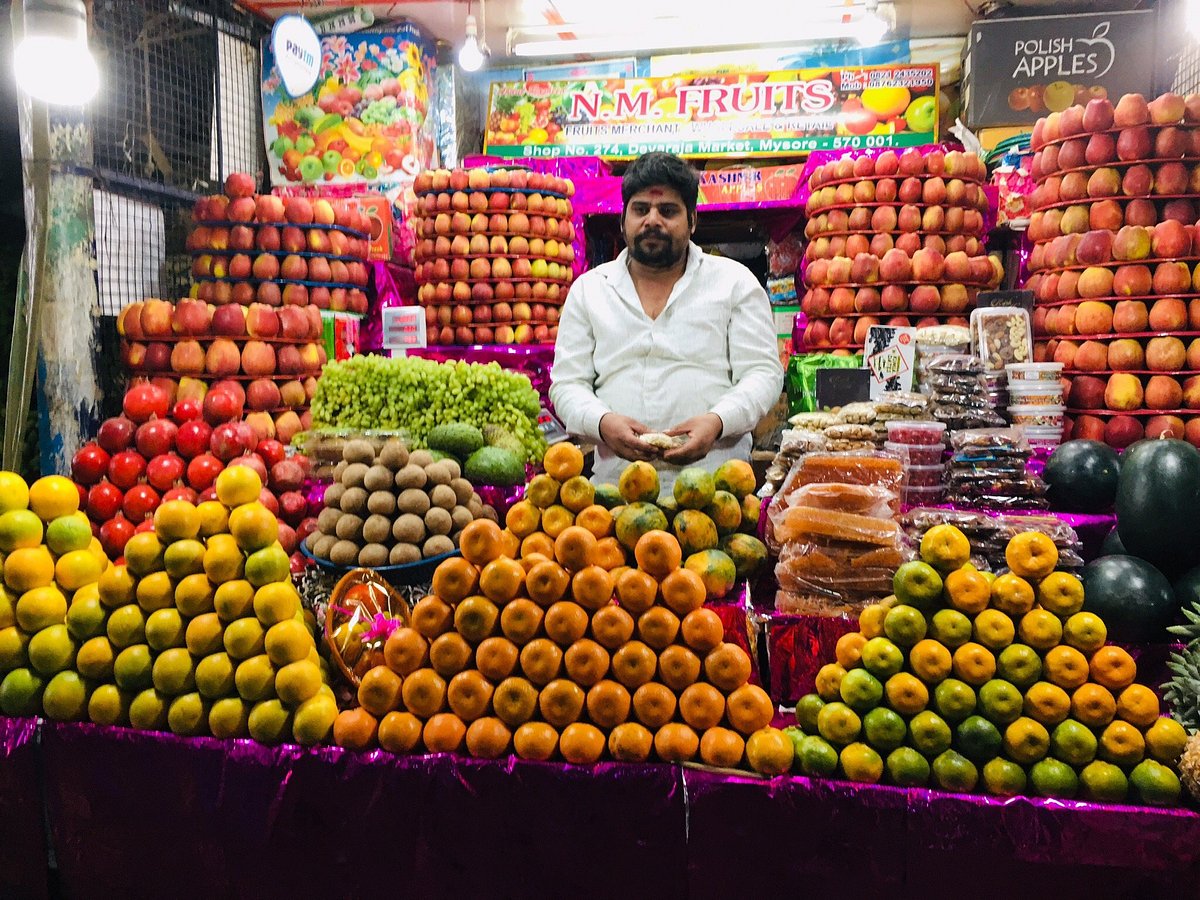In this vibrant photograph, an Indian fruit merchant with a black goatee and a puffy hairstyle stands proudly amidst his colorful display at Shop No. 274, DAVARAJA Market in Mysore, India. He wears a white button-down shirt and is surrounded by carefully stacked piles of fruit, forming partial pyramids owing to some missing pieces. The fruits, consisting of oranges, lemons, apples, and possibly papayas and limes, create a rich tapestry of colors including light green, orange, yellow, red, pink, tan, and black. Behind him, a sign reads "N.M. Fruits" with "Fruits Merchant" plainly visible in smaller lettering below. This bustling marketplace scene is further detailed by an additional sign mentioning "Polish Apple" and "57001". The fruit is elegantly presented both in front of and behind the merchant, who stands at the center, ready to serve his customers.